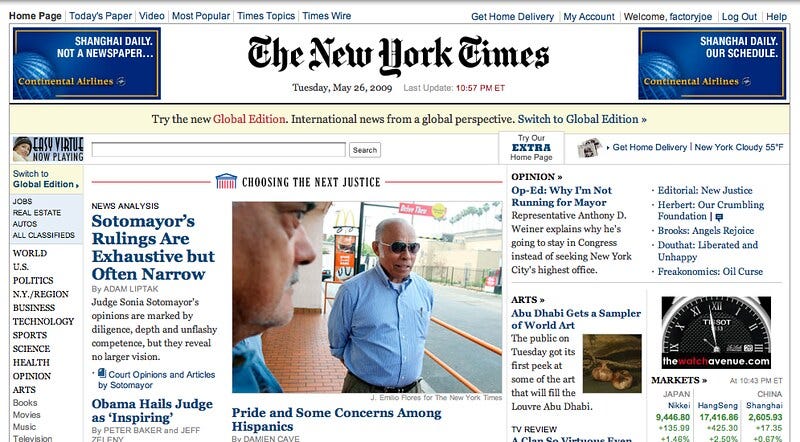Headline of the New York Times newspaper reads, "Choosing the Next Justice," under the section "News Analysis." The central article, authored by Adam Liptack, is titled "Sotomayor's Rulings Are Exhaustive but Often Narrow." It discusses Judge Sonia Sotomayor's judicial opinions, characterizing them as marked by diligent depth and unflashy competence, yet lacking a broader vision.

Included in this coverage is a court opinion piece by Judge Sotomayor herself, capturing her views and judicial approach. Additional related articles include "Obama Held Judge as Inspiring," by Peter Baker and Jeff Zeleny, and "Pride and Some Concern Among Hispanics," by Damian Cave, which explore the broader implications and community reactions to her nomination.

On the right-hand side of the page, under the "Opinion" section, an Op-Ed piece titled "Why I'm Not Running for Mayor" by Representative Anthony D. Weiner explains his decision to remain in Congress rather than pursue New York City’s mayoral office.

In the "Arts" section, an article highlights a public preview held on Tuesday of art that will be featured in the forthcoming Louvre Abu Dhabi, describing it as a global sampler of world art.

The "Editorial" section contains a piece labeled "New Justice," presumably offering the newspaper’s official stance or thoughts on the impending nomination and its significance.